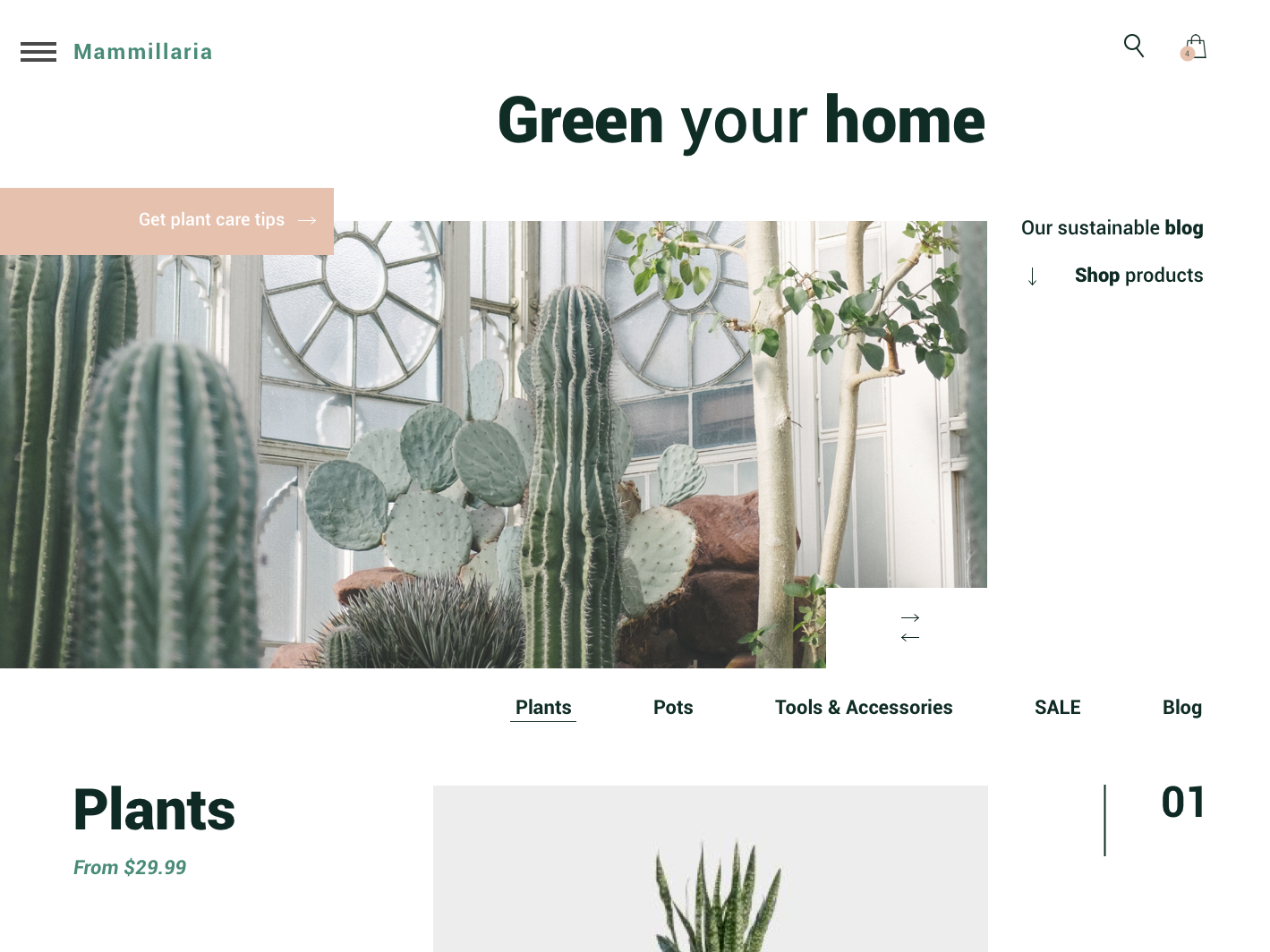This is a detailed screenshot from a company’s website that specializes in selling potted plants. 

In the top left corner, there are three horizontal lines stacked atop each other, presumably indicating a menu icon. The brand name "Mammalaria" is displayed prominently beside it. The top right corner features a magnifying glass icon for search functionality and a shopping bag icon with a number "4" overlay, possibly indicating items in the cart.

Centrally placed and in larger, bold text, the phrase "Green Your Home" stands out. Just below this, to the left, there's a photograph showcasing various plants, including several types of cacti, set against a backdrop featuring stylized windows and additional plant varieties, such as a small tree. An overlay in the top left of this picture reads "Get Plant Care Tips."

To the right of this photograph, there are links labeled "Our Sustainable Blog" and "Shop Products." Beneath the photo, there is a navigation bar with five options: "Plants" (which is underlined, indicating it might be the current selection), "Pots," "Tools & Accessories," "SALE" (in all caps to grab attention), and "Blog."

In the bottom left corner of the page, bold black text against a white background announces "Plants from $29.99." Moving towards the middle of the page, there's another photograph, although it is partially cut off by the page's end. This image captures the top spiky portion of a green plant but does not include the pot or the rest of the plant. To the right side of this partial image, there is a number "01."

Overall, the screenshot provides an engaging preview of the company's offerings and navigation options, focusing on plant variety, pricing, and additional resources such as plant care tips and a blog.